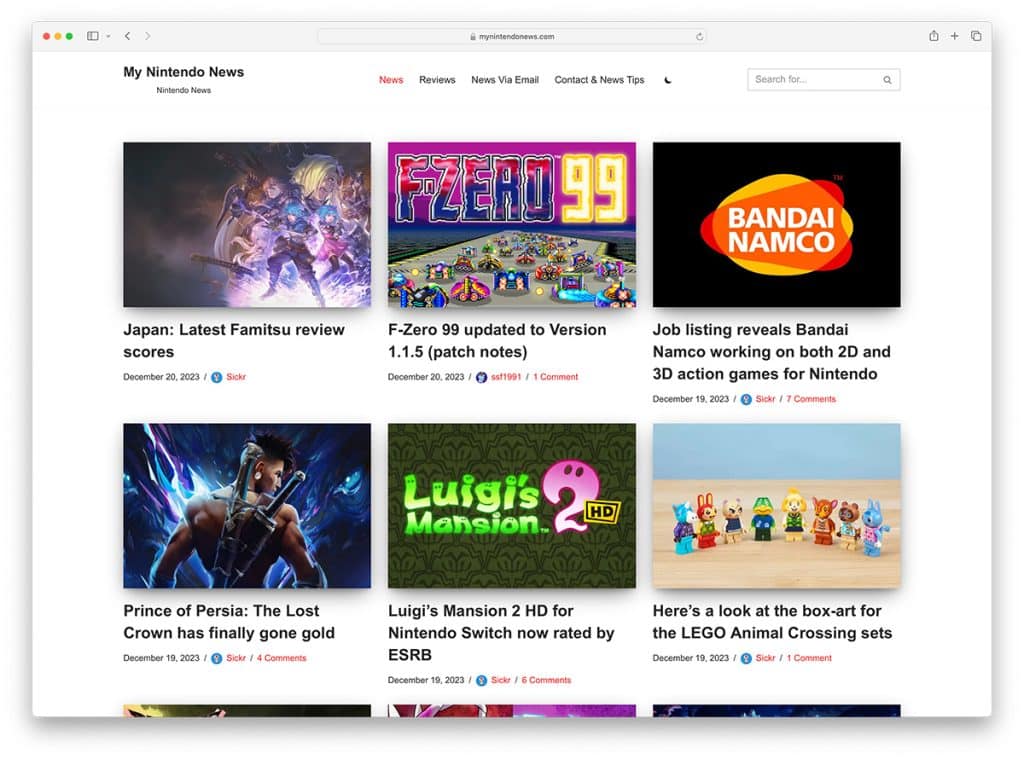This appears to be a description of a screenshot from a webpage, possibly a gaming news or reviews site. Here's a cleaned-up and detailed caption:

---

A detailed screenshot of the Mynintendonews.com webpage, showcasing its colorful navigation bar with red, yellow, and green sections, including a left arrow. The site header includes links for news, reviews, contact information, and a search bar. Current highlights include Japan's latest pharmacy review scores from December 20, 2033, and an update to version 1.5 of CSO99. Thumbnail images suggest a variety of articles - reviews of Bandai Namco's 2D and 3D action games for Nintendo, including a new title, "The Super Trilogy of the Lost Kings," which received a gold rating. Featured prominently in the snapshot is a rear shot of the Prince of Persia character brandishing dual swords, a comparison showing Luigi's Mansion 2 as more affordable than a Nintendo Switch, and a first look at the box art for the LEGO Animal Crossing sets, dated December 10, 2023, all set against a clean, white background.